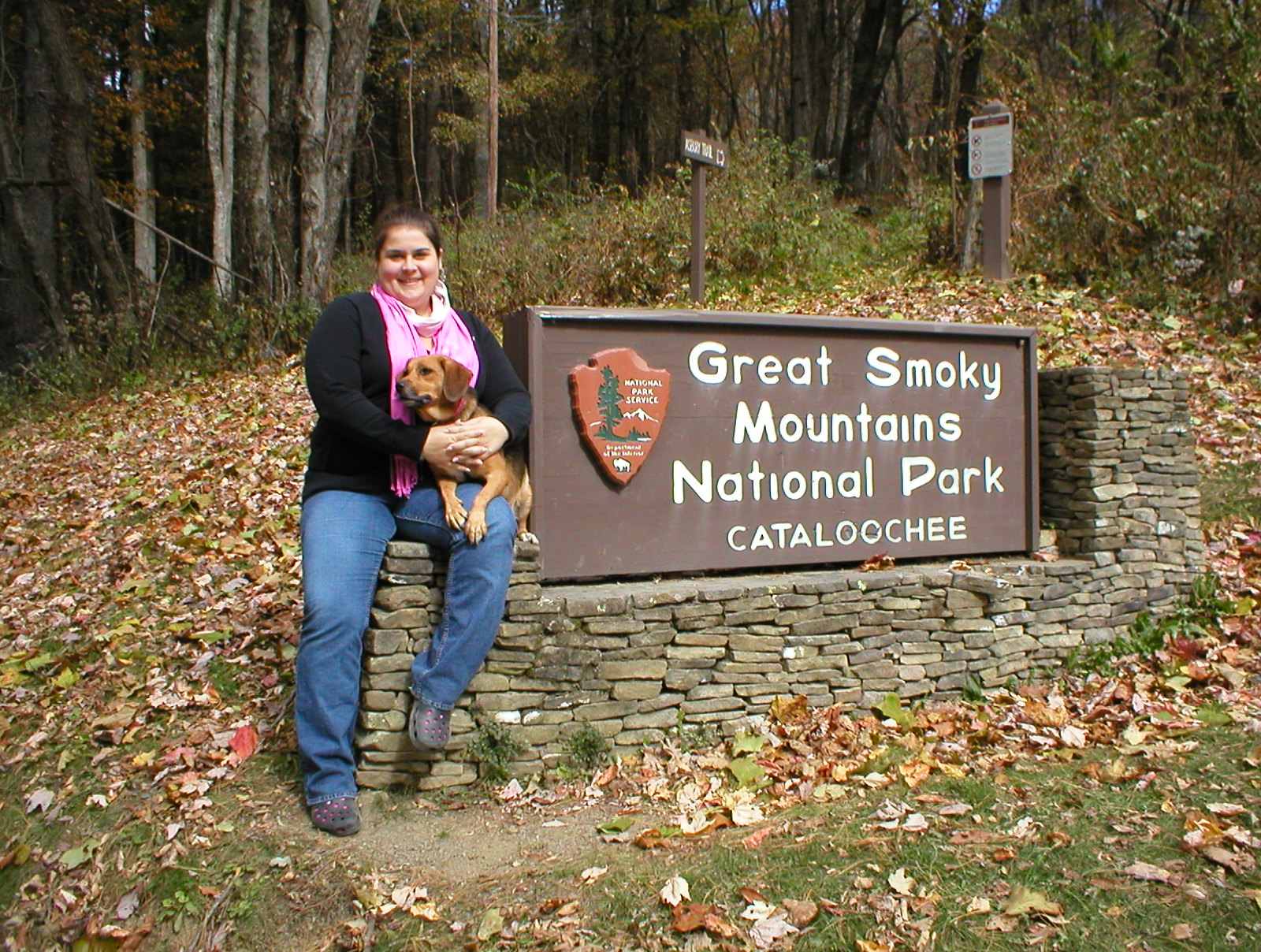In this vibrant photograph, a cheerful young woman, likely in her 20s, is sitting on a stone wall adorned with the Great Smoky Mountains National Park, Cataloochee sign. The woman has her hair pulled back and is dressed in blue jeans, hiking shoes, a pink shirt, and a layered cardigan—reddish with a blackish tinge. She holds a small, brown dog comfortably on her lap, somewhere between the size of a beagle and a small lab. Behind her, the landscape shifts into a wooded area, with a hill covered in crunchy, fallen leaves of brown, yellow, and red hues, leading up to a dense forest of tree trunks. Above the main sign, which is brown with white graphics, are a couple of unreadable smaller signs and an orange, shield-shaped emblem typical of National Park signage. The woman's bright smile and relaxed posture suggest she is enjoying a peaceful moment in this picturesque national park setting.